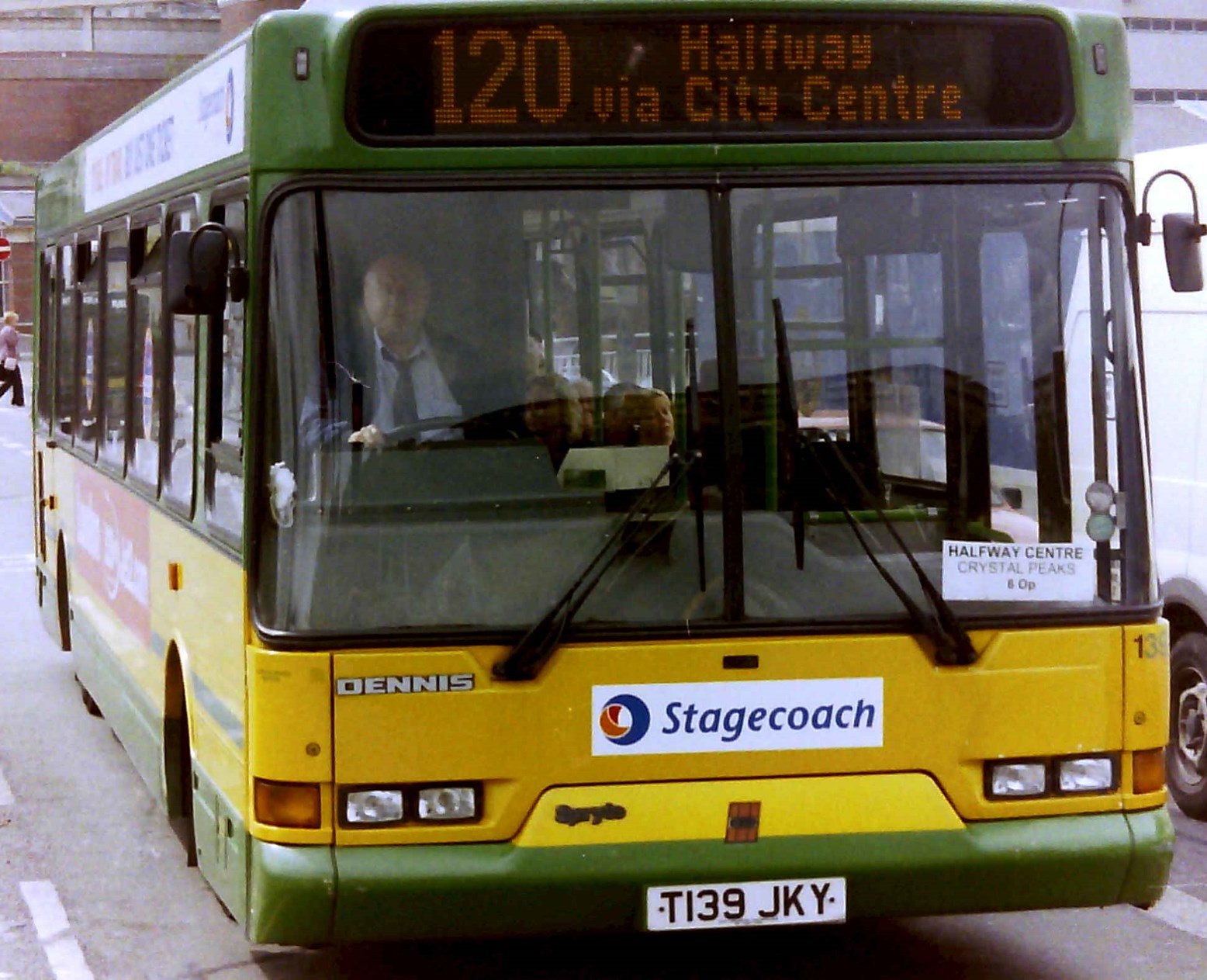This image captures a close-up view of a Stagecoach Dennis bus, positioned centrally and parked, identifiable by its license plate "T139 JKY." The bus prominently displays a light-up text reading "120 via Halfway City Center," and there's a paper placard that says "Halfway Center Crystal Peak." The bus features a design with a green top and bottom, while the main body is honey yellow, accented by orange text and some black elements. The driver, situated on the right side of the bus, is wearing a blue jacket, a black tie, and has his top shirt button undone. Visible through the bus windows are passengers seated behind the driver. In the top left corner of the image, part of a red brick building can be seen, with the gray road stretching out beneath the bus. The overall setting appears to be a typical urban scene, possibly captured by a commuter or passerby.